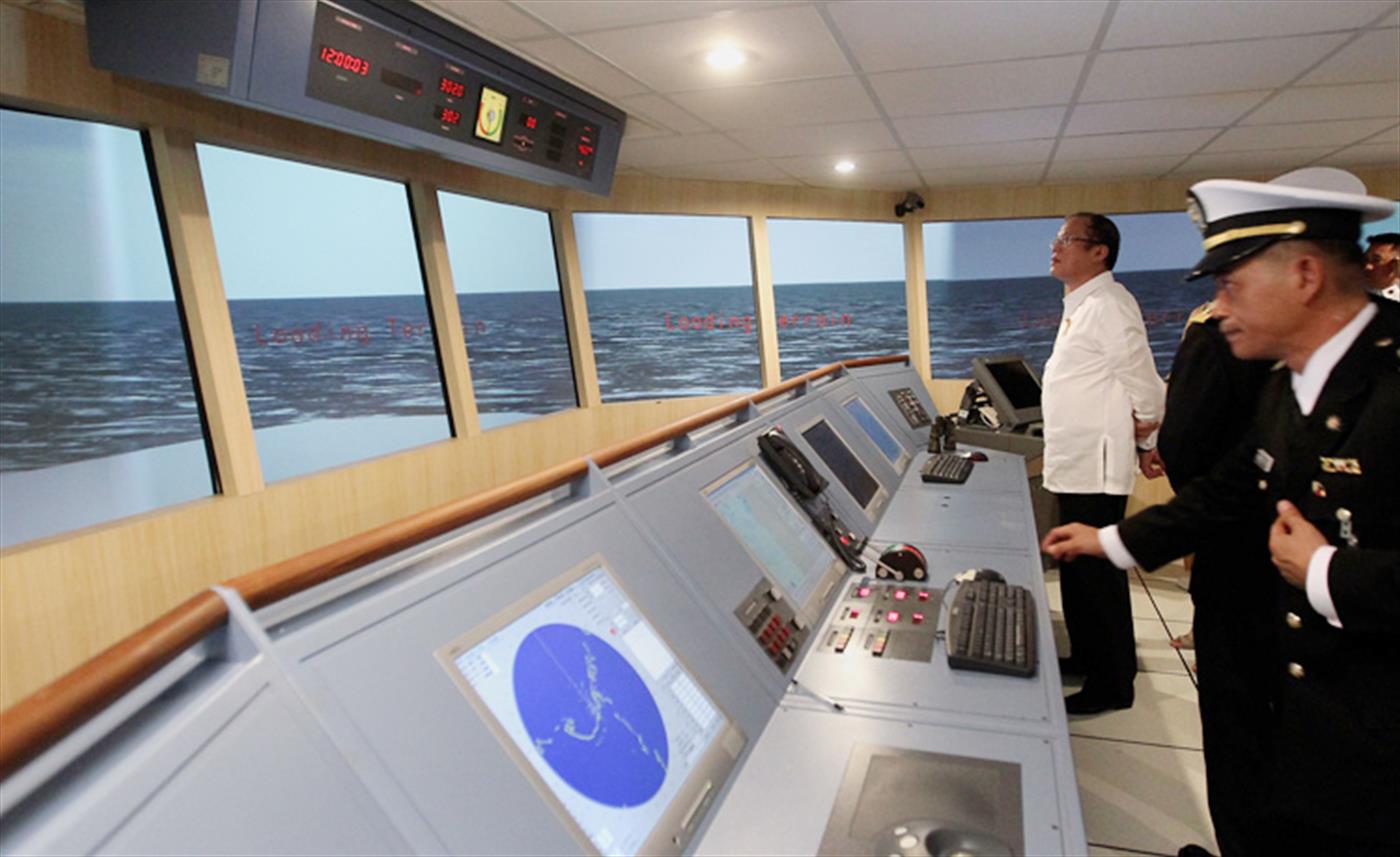This landscape photograph captures the bustling control bridge of a ship, where several officers, including the captain, diligently oversee the vessel's navigation. The cabin's white drop ceiling, embedded with lights, adds clarity to the space. Large, panoramic windows, numbering seven to nine, provide a sweeping view of the vast, beautiful blue sea and lighter blue sky, showcasing the ship's ongoing voyage. Dominating the top left of the image is a piece of machinery colored in blue and black, displaying red digital numbers. Centrally located is a touchscreen panel with yellow, green, and red indicators, contributing to the array of grey instrument panels, Doppler radar screens, and numerous lighted red buttons. The scene also features a silver table strewn with keyboards, a mouse, a phone, and additional screens. Closest to the viewer in the bottom-left corner stands the captain, recognizable by his black uniform adorned with medals and a black, white, and gold captain's hat. Behind him, another officer can be seen in a similar uniform, while farther in the background, a man in a white shirt and black pants is attentively monitoring the control panels.